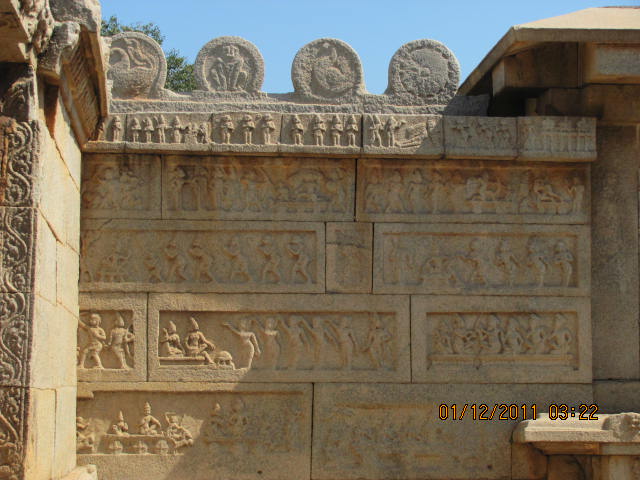The image depicts an ancient stone wall adorned with intricate carvings, suggestive of a historical site in a warm country possibly in Asia or South America, potentially linked to the Mayan or Aztec civilizations. The artwork on the wall features an array of human figures engaged in various activities, such as dancing or hunting, telling what appears to be a story through these detailed engravings. Each stone block varies in size and houses different male and female figures, meticulously chiseled into the tan and rust-textured surface. At the top of the wall, three large circular stone sculptures with carved patterns stand out. The background showcases a clear, bright blue sky with the top of a leafy green tree peeking in from the left side. A timestamp in orange text with a black border at the bottom right corner reads "01/12/2011 03:22," indicating a possible tourist photograph capturing this popular attraction.